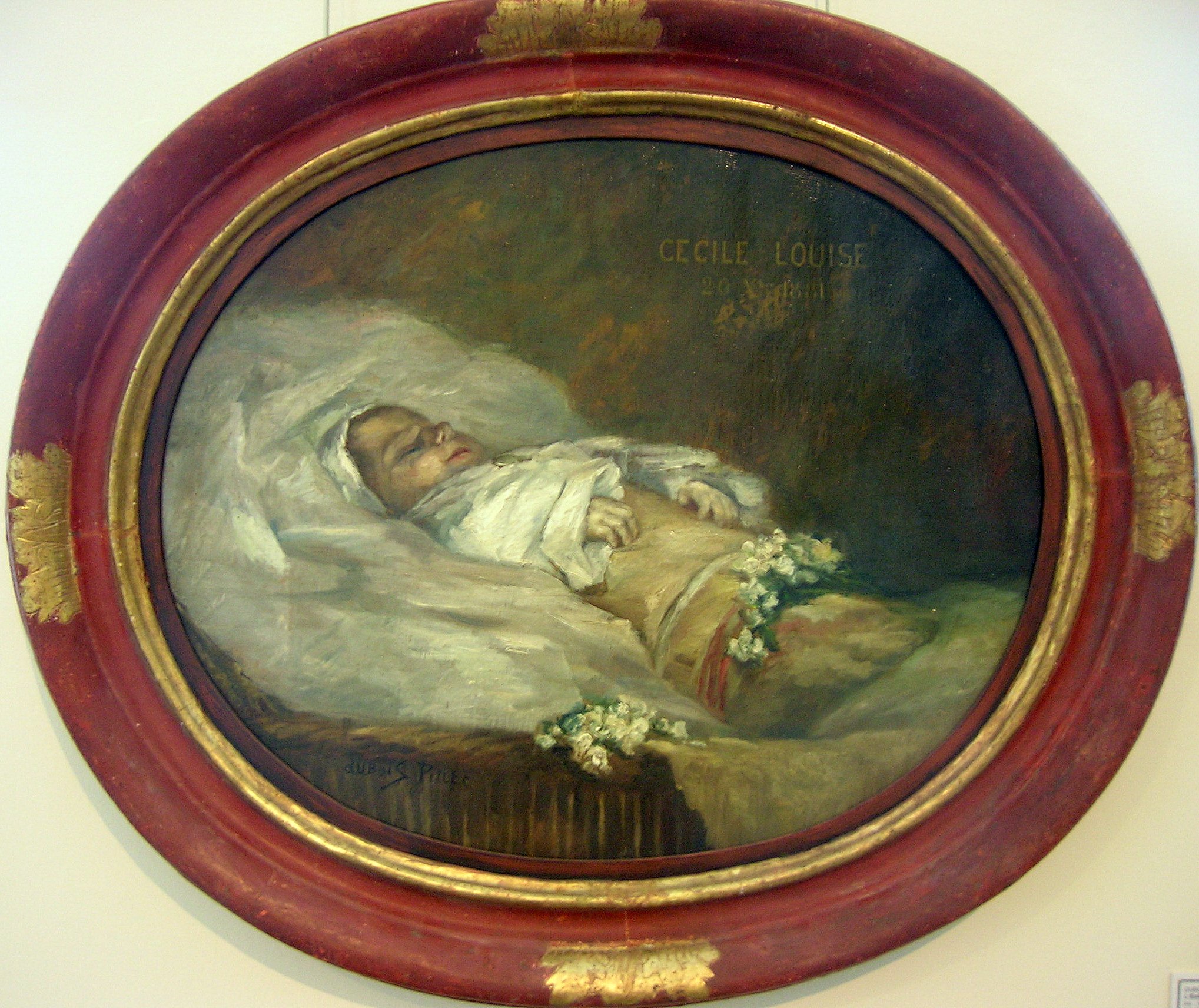In the image, an oval-shaped painting hangs on a white wall in a well-lit environment. The painting is horizontally oriented, longer width-wise, and enclosed in a red frame adorned with gold leafy trim at the four extreme points of the oval. The frame features several layers of trim, including a gold band on the inner side and a flat red part flush with the canvas. The painting itself depicts an infant, possibly deceased, lying in what appears to be a bassinet or a baby coffin, adorned with white cloth and floral decorations. The child, identified as Cecile Louise by an inscription on the canvas, is dressed in a white top with its belly, hands, and face partially exposed, seemingly peaceful with eyes closed and wearing a white bonnet. The background features dark, ominous shades of green and brown, contrasting with the bright, serene appearance of the baby in the foreground. The main colors in the painting are green, yellow, and white.